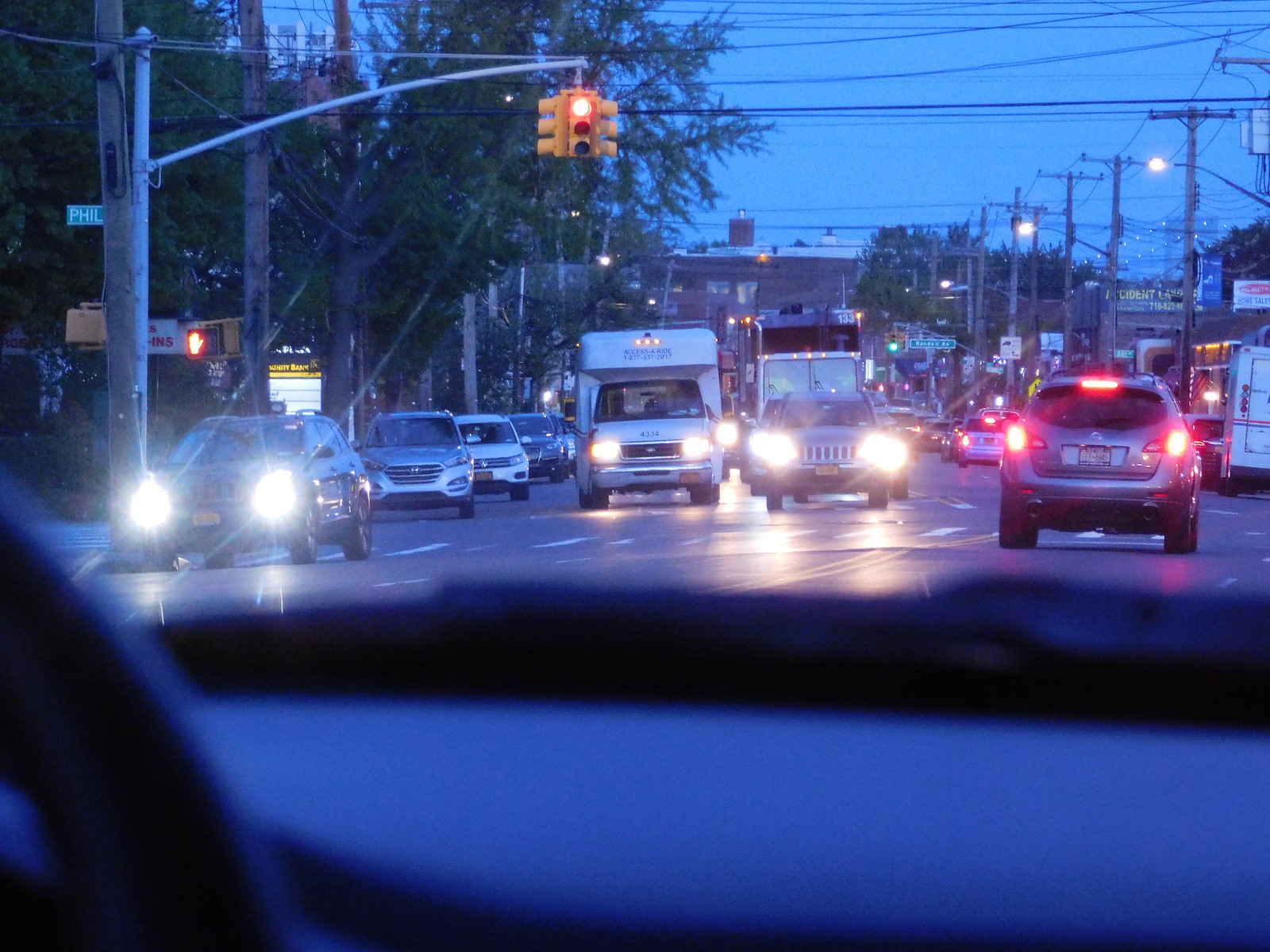This color photograph captures a low-light road scene viewed from inside a car. Dominating the bottom left corner is a blurred section of a steering wheel and dashboard in dark blue, framing the dimly lit road ahead. The dark blue asphalt stretches into the distance, under a similarly dusky blue sky. Ahead, the road is occupied by several vehicles, including a prominent white van and a car, both with headlights beaming directly toward the viewer. Numerous additional cars can be seen in the left lanes, also illuminated by headlights as they travel towards us. 

In the right lane, a silver car is moving away, its red tail lights clearly visible against the night. Overhead, power lines stretch across the scene toward the left, paralleled by a series of street lights. Tree branches creep into the top right corner, adding to the silhouetted landscape. In the distance to the left, street signs are faintly visible, adding a sense of depth to the composition. A set of traffic lights hangs over the street, encased in a yellow box, with the amber light glowing at the top, signaling a moment of caution in the otherwise steady flow of night-time traffic.